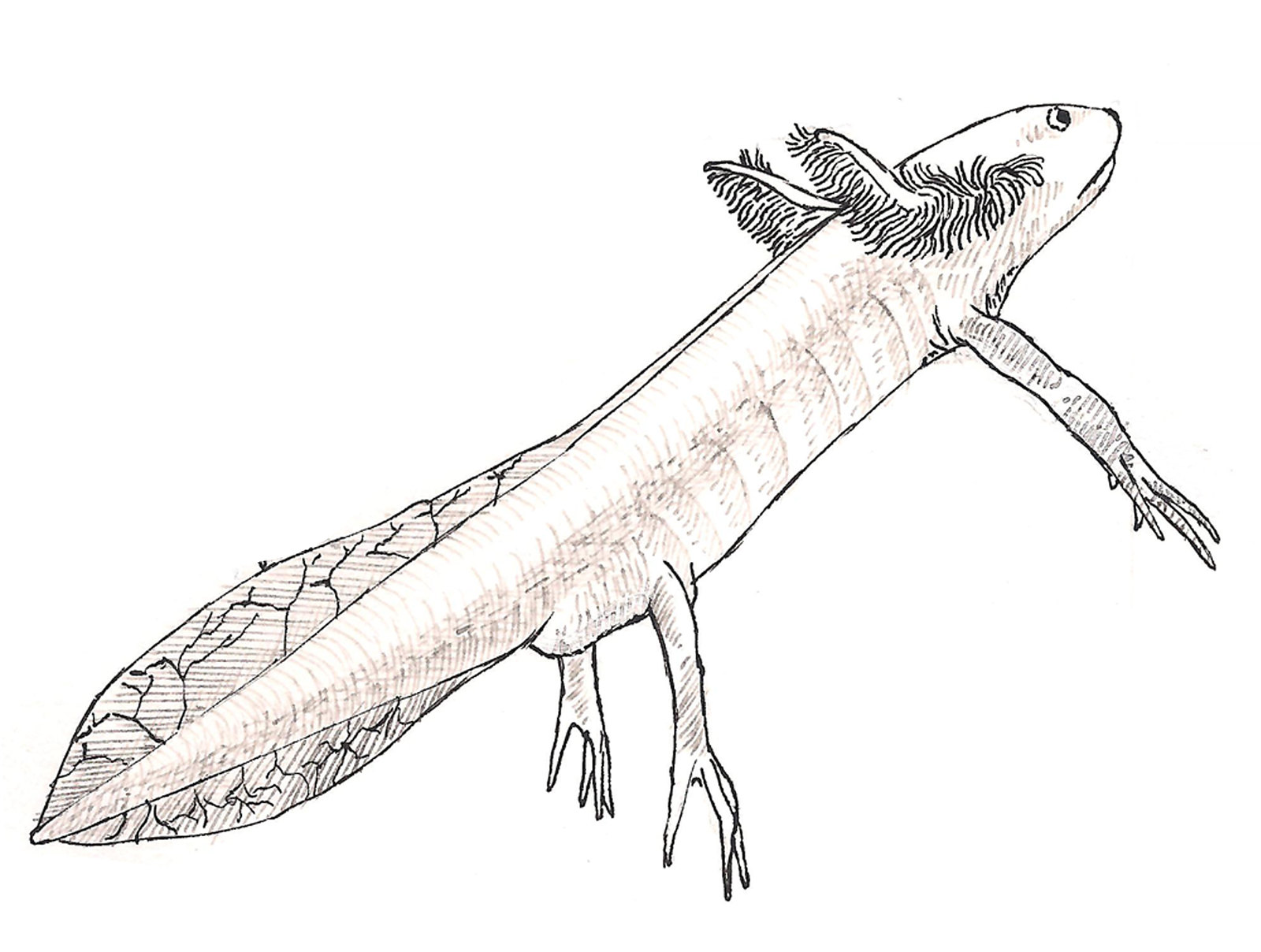This image features a cartoonish, hand-drawn depiction of a young salamander or tadpole-like creature, prominently set against a stark white background. The creature inclines from the bottom left to the top right of the image. Outlined in black and shaded with a primarily brown hue, the drawing has some pinkish tones blended into its body. This whimsical animal, seen in a side view, exhibits a unique combination of features: it has a glum expression with straight-lined mouth, large eyes, and peculiar antler-like cilia emanating from its ears. Its anatomy includes four legs, though only three are visible, with the rear pair showing four fingers each and the front leg presenting five fingers. Detailed lines depict veins running along its tail, suggesting a mix of anatomical accuracy and imaginative elements.